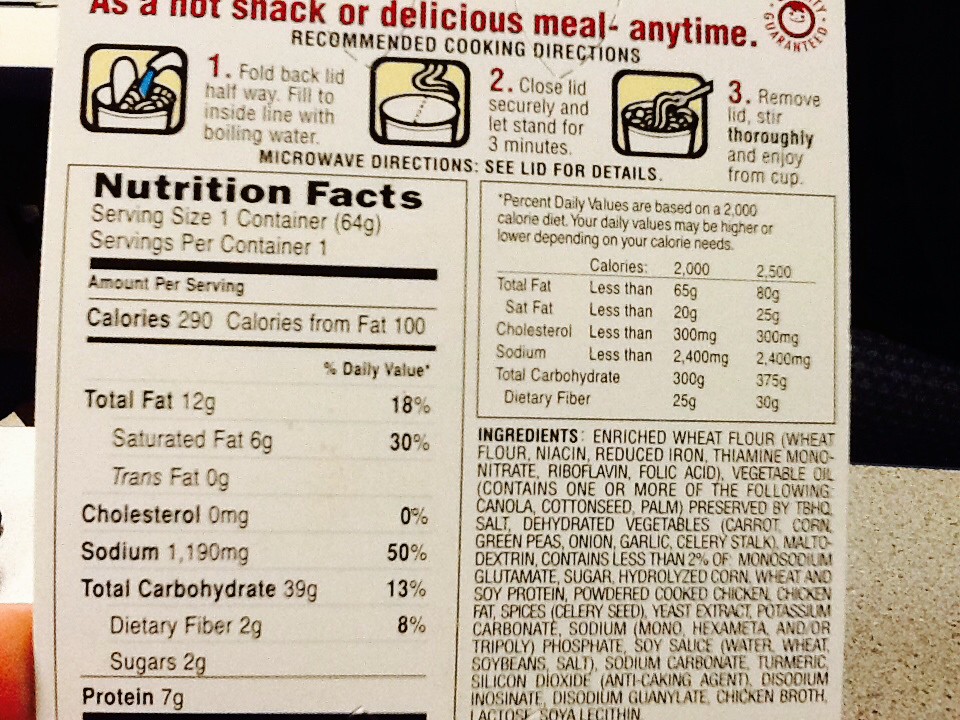A close-up image of a nutrition label on the back of a cup of instant noodles reveals details about its nutritional content and preparation instructions. Marketed as a convenient hot snack or a delectable meal at any time, the product's packaging features a three-step preparation guide: fold the lid halfway, add boiling water, close the lid and let it steep for three minutes, and then stir before enjoying. Nutritional information indicates the serving has 290 calories and contains 7 grams of protein. The fat content is significant with 30% coming from saturated fats. There are also 39 grams of carbohydrates, which include dietary fiber and sugars. Notably, the product is free from cholesterol.